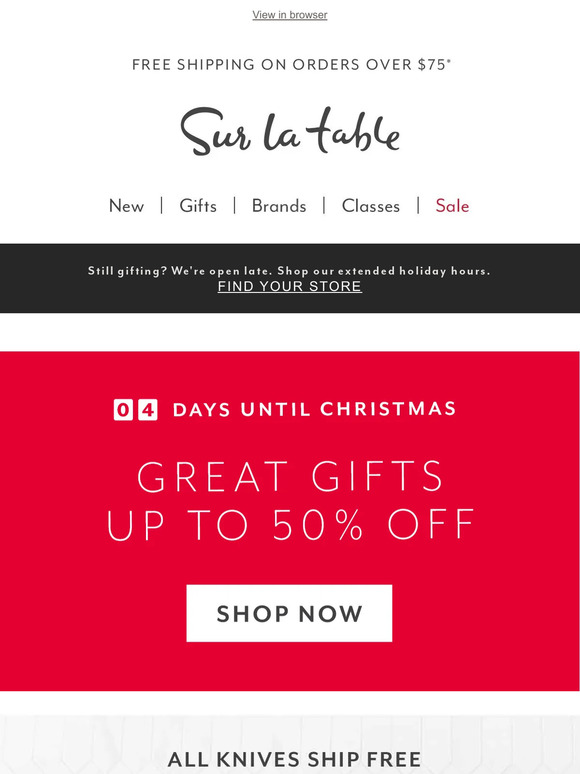This image is a screenshot from a mobile device. At the very top, there's an underlined text link that reads "View in Browser," indicating an option to view the content in a web browser. The upper section of the image has a white background with the text: "Free shipping on orders over $75 for Sur La Table." Below this, four clickable links read "New Gifts," "Brands," "Classes," and "Sale."

A black rectangular bar follows, containing a clickable link that says "Find Your Store," directing users to locate a nearby store. Adjacent text promotes extended holiday hours with the phrases "Still gifting?" and "Open late. Shop our extended holiday hours."

Further down, a prominent red box displays the message "Four days until Christmas" and "Great gifts up to 50% off," accompanied by a white "Shop Now" button in the center.

The image ends with another section starting to appear, featuring dark gray block letters on a white background, proclaiming "All knives ship free." The full content of this section is not visible in the screenshot as further scrolling is required. The ad is for Sur La Table, a kitchenware retailer.